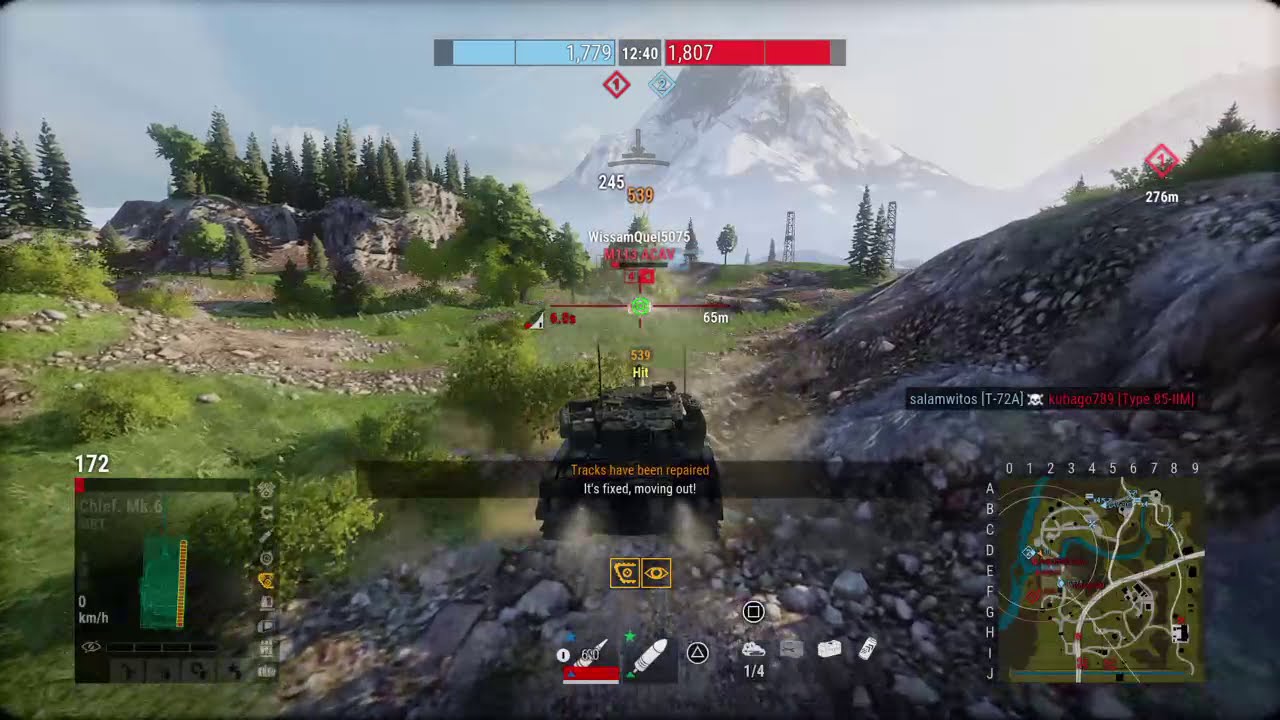This screenshot captures a moment in a tank-focused video game. The scene, set against a backdrop of a snowy mountain, unfolds in a European-like landscape featuring lush evergreens and rocky granite hills. Front and center, the player's green tank is advancing forward, emitting exhaust plumes, and navigating through a terrain scattered with rubble and bushes. The left side of the image includes grass interspersed with dirt trails and additional granite features, while a prominent rocky hill adorned with trees rises in the left background.

On the game's interface, several details enhance the gameplay experience. The bottom left corner displays the tank's health indicator in green, with accompanying buttons and yellow text. Centrally aligned below the tank are various weapon selection options, while the bottom right hosts a mini-map showing the battlefield. The top section of the screen reveals scores of 1,779 for the blue team and 1,807 for the red team, spotlighting an ongoing competitive match. Additional elements on the HUD include speed stats, control icons, and a red symbol marking a location 27.6 miles away. The entire image, despite its somewhat low resolution, effectively conveys the immersive and strategic environment of this military-themed game.